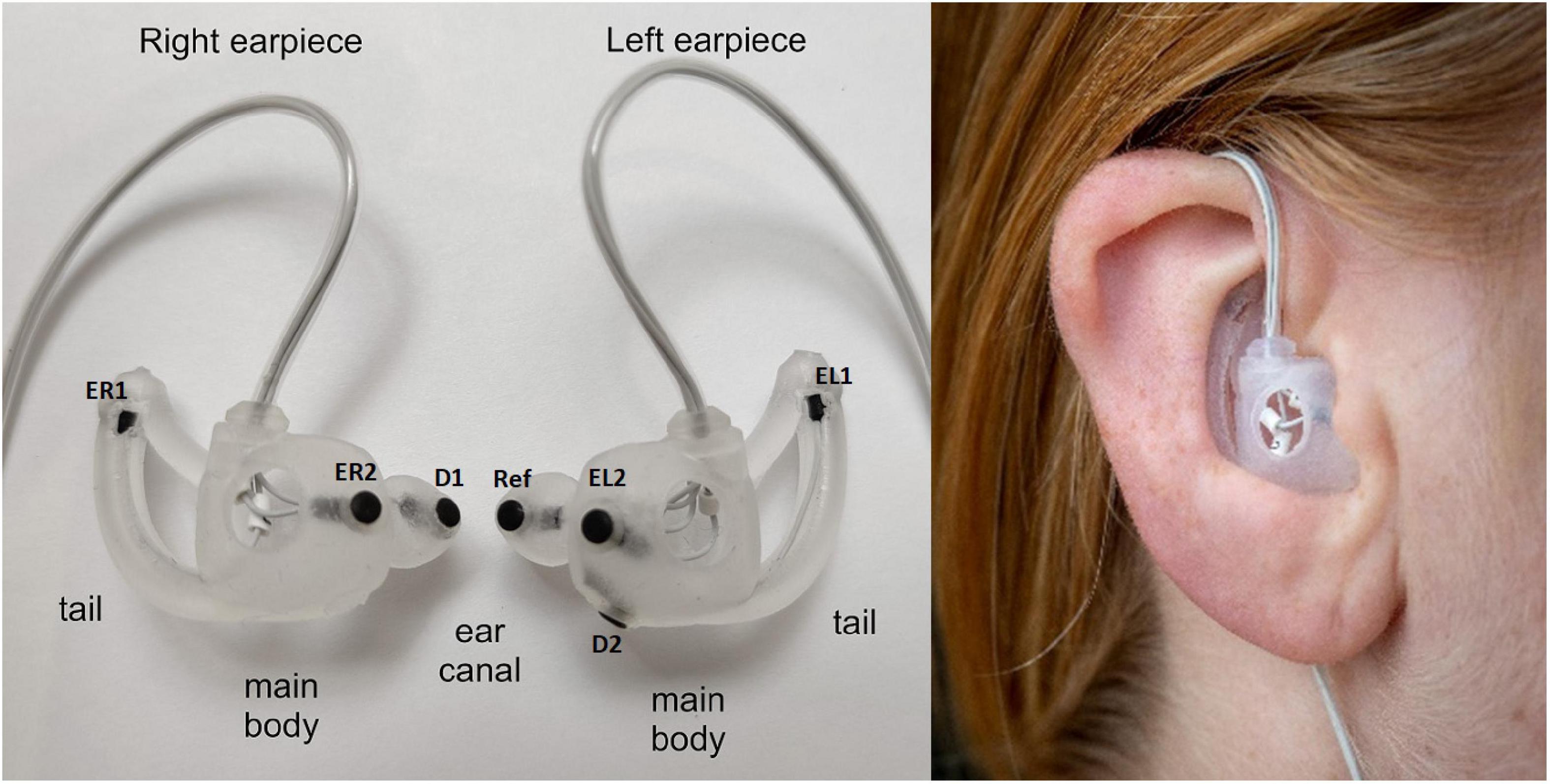The image is a detailed two-part diagram of a cochlear implant or hearing aid. On the left, the diagram displays a transparent or milky white implant, labeled meticulously with terms such as "tail," "main body," "ear canal," "ER1," "ER2," "D1," "REF," "EL2," and "EL1." Additionally, the text in black at the top of the left diagram denotes "right earpiece" and "left earpiece," describing the components connected by a thin wire. On the right side of the image, an individual with long reddish-brown hair is shown wearing the implant. The device is small and inserted into the ear, with the wire wrapping over the top and the tail portion extending behind and below the ear after curving around it.